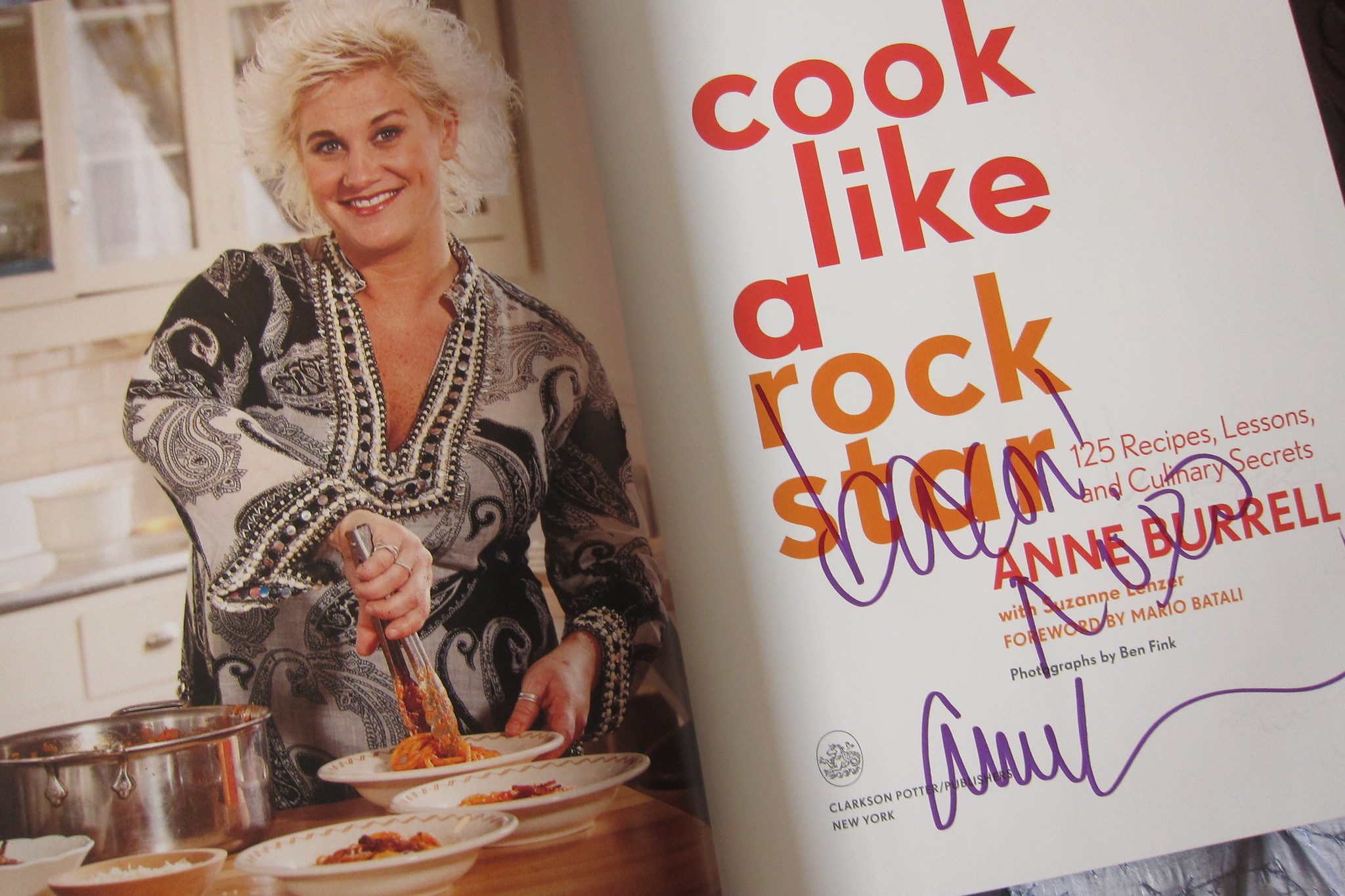The image depicts an open cookbook. The left page features a vibrant photograph of a Caucasian woman in her 30s with voluminous, fluffy blonde hair, wearing a long-sleeved, black-and-white blouse. She is smiling at the camera while standing in a kitchen, holding tongs and serving spaghetti with red sauce onto plates from a large silver pot on the table in front of her. Behind her, kitchen cabinets are visible, adding to the culinary ambiance. The right page of the book displays the title in bold red and orange text: "Cook Like a Rockstar: 125 Recipes, Lessons, and Culinary Secrets" by Anne Burrell with Suzanne Lenzer, foreword by Mario Batali, photographs by Ben Fink, published by Clarkson Potter. There is a handwritten signature in purple marker reading "Bacon XOXO Anne."